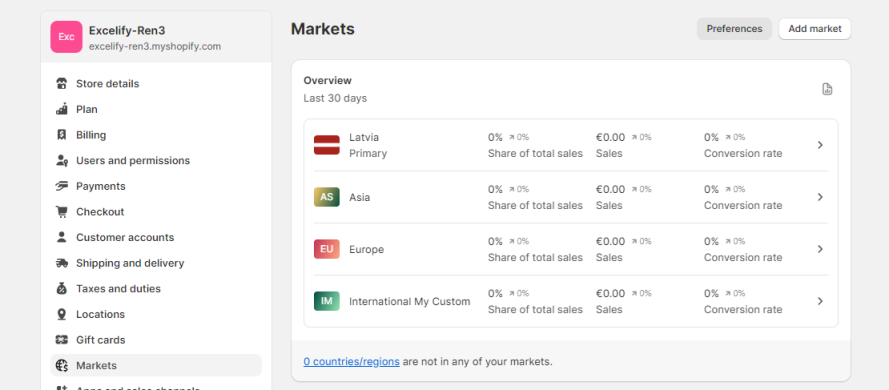The screenshot captures the Shopify account of the user named Excelify-Ren3, showcasing their efforts to track and manage various markets. The interface presents a comprehensive layout with a detailed left sidebar featuring multiple tabs: Store Details, Plan, Billing, Users and Permissions, Payments, Checkout, Customer Accounts, Shipping and Delivery, Taxes and Duties, Locations, Gift Cards, and Markets. Each tab is accented with its own unique icon for easy navigation.

The focus of the screenshot is on the 'Markets' tab, which is currently expanded on the right side of the panel. The Markets overview provides a summary of the last 30 days, highlighting different regions like Latvia (noted as the primary market with its own icon), Asia, Europe, and International Custom. At the bottom of this section, blue text indicates that "0 countries and regions are not in any of your markets." The display includes detailed metrics such as the share of total sales from each market and conversion rates.

In the top-right corner of the interface, two prominent buttons are visible: one for 'Preferences' and the other for 'Add Market,' offering quick access to further customization and expansion of market strategies. This screenshot exemplifies a structured approach to ecommerce management through Shopify's versatile platform.